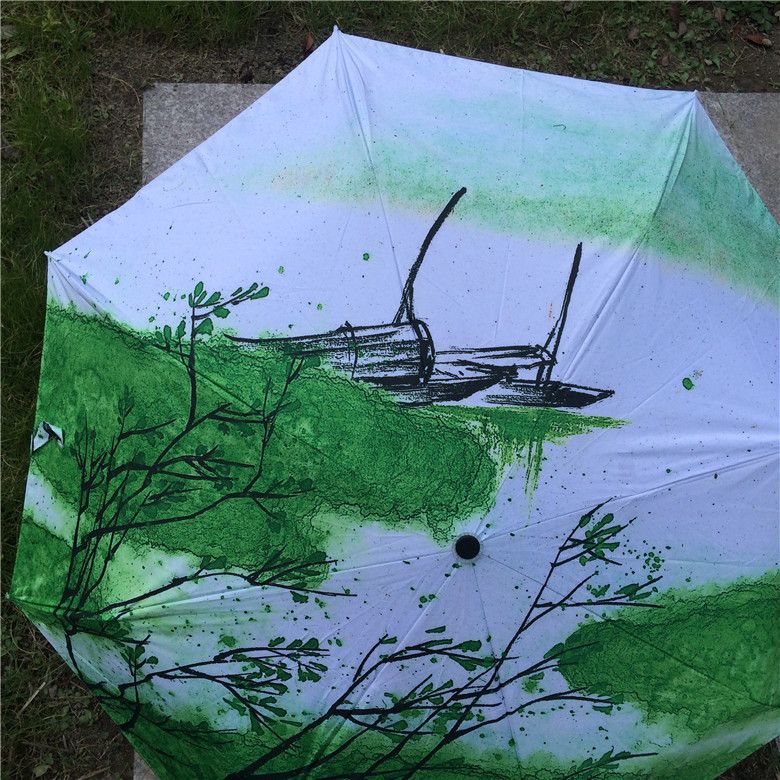The image depicts a custom-designed white umbrella adorned with an intricate black sketch of a building in the middle, partly obscured by branches adorned with small leaves. The branches extend outward, intermingling with splashes of green that mimic foliage, creating an impression of blending with the natural environment when viewed from above. The umbrella seemingly lies on a piece of concrete amidst green grass and some dirt in what appears to be a park setting. Despite its artistic design, the umbrella appears somewhat worn and discarded. A black signature in the bottom right corner identifies its origin, likely from dhgate.com, promoting the UniNature umbrella. The black central hub where the umbrella's spokes converge is also noticeable.